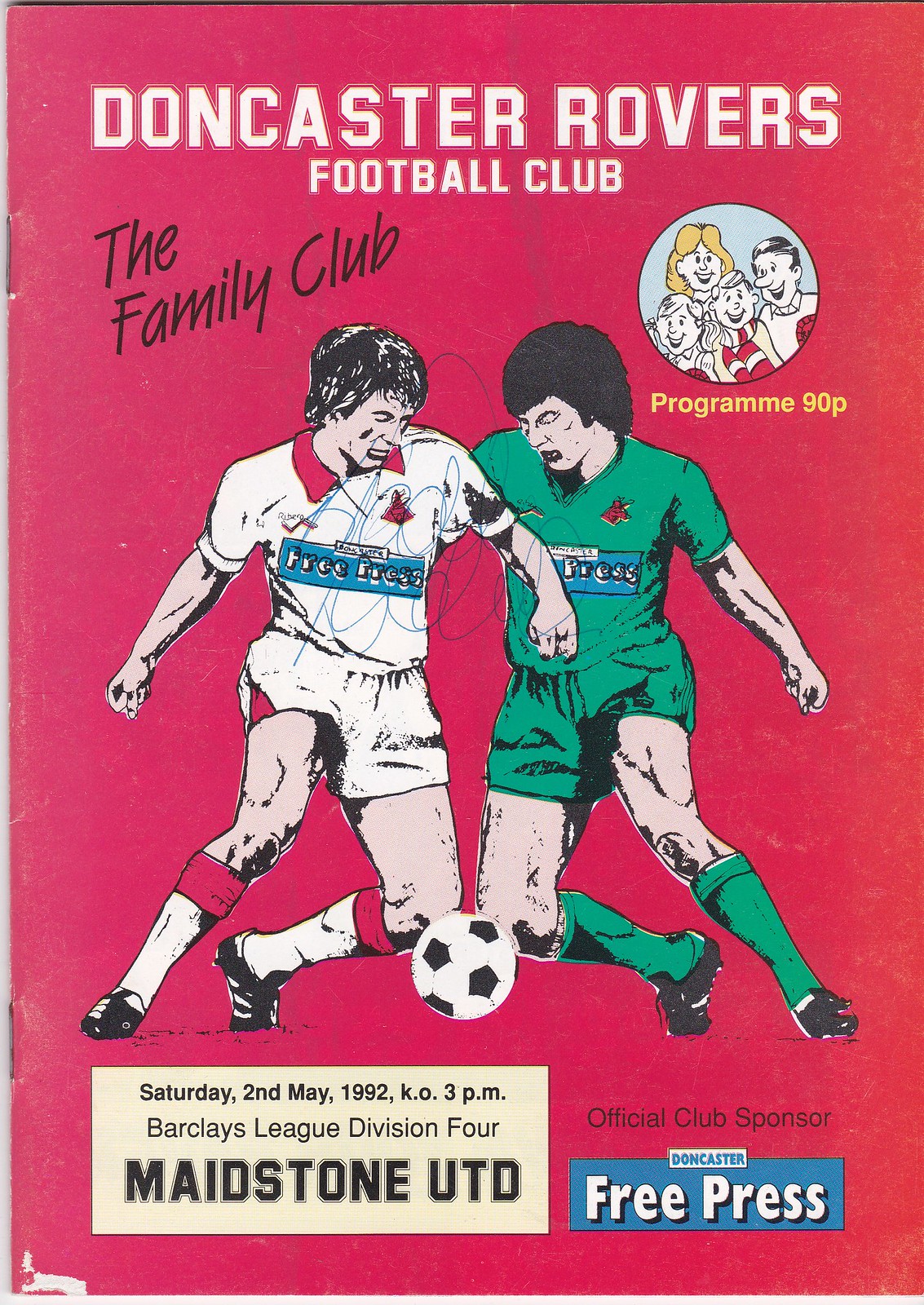This is an image of a program cover for the Doncaster Rovers Football Club. The background is entirely red, with white letters at the top stating "Doncaster Rovers Football Club" and to the left in black letters, it says "The Family Club." To the right, a blue circle contains cartoon drawings of a family: a woman with blonde hair, a man, and two children standing in front of them. Below this image, in yellow letters, it reads "Program 90p." 

In the center, there are illustrated drawings of two soccer players positioned around a black and white soccer ball. The player on the left is wearing an all-white jersey with red details, while the player on the right dons a green jersey. Both have "Free Press" displayed in a blue box on their shirts. At the bottom of the program, a yellow box states "Saturday 2nd May 1992 Barclays League Division 4." Additional text in the lower left corner mentions "KO 3 p.m. Maidstone UTD," while the lower right corner includes "Official Club Sponsor: Doncaster Free Press."